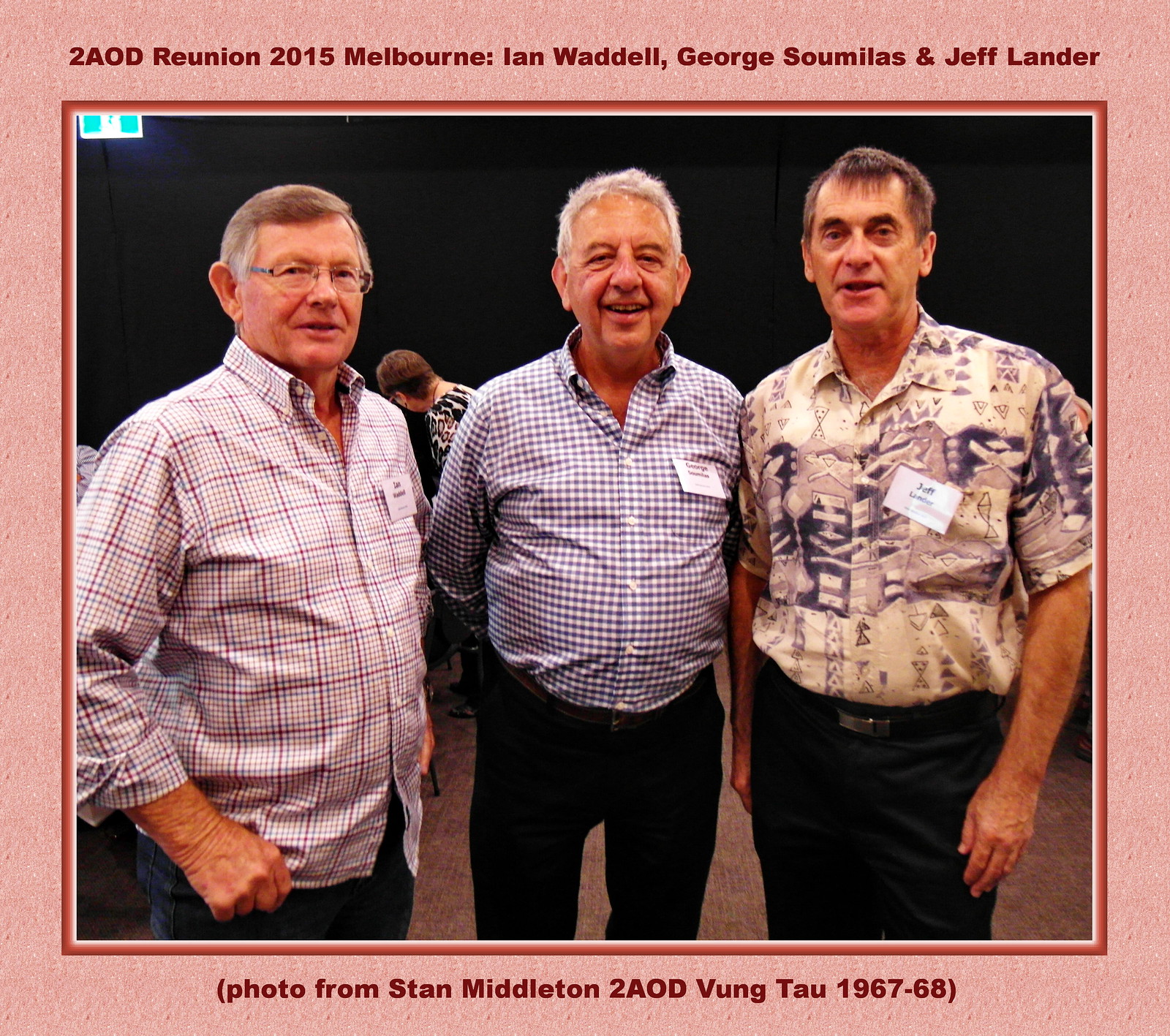In this detailed photograph, three elderly gentlemen are standing side by side, each wearing a button-down shirt and dark pants. The man in the middle is smiling warmly, dressed in a plaid blue shirt with dark pants and sporting gray hair. To his right stands a slightly younger man wearing glasses and a red and pinkish plaid shirt, with brown hair beginning to gray at the sides. On the left, the third man has dark hair and dark eyes, clad in a uniquely designed shirt and dark pants. All three men have name tags pinned to their shirts, with the men on the left and middle wearing long sleeves, while the man on the right is in a short-sleeved shirt. The background features a black backdrop and a brown carpeted floor. Encasing the photograph is a digitally generated light pink or salmon pink border with a grainy texture. At the top of the border, the text reads: "2AOD Reunion 2015 Melbourne, Ian Waddell, George Somilas, and Jeff Lander." The bottom text in parentheses states: "Photo from Stan Middleton, 2AOD Vung Tau, 1967-68."